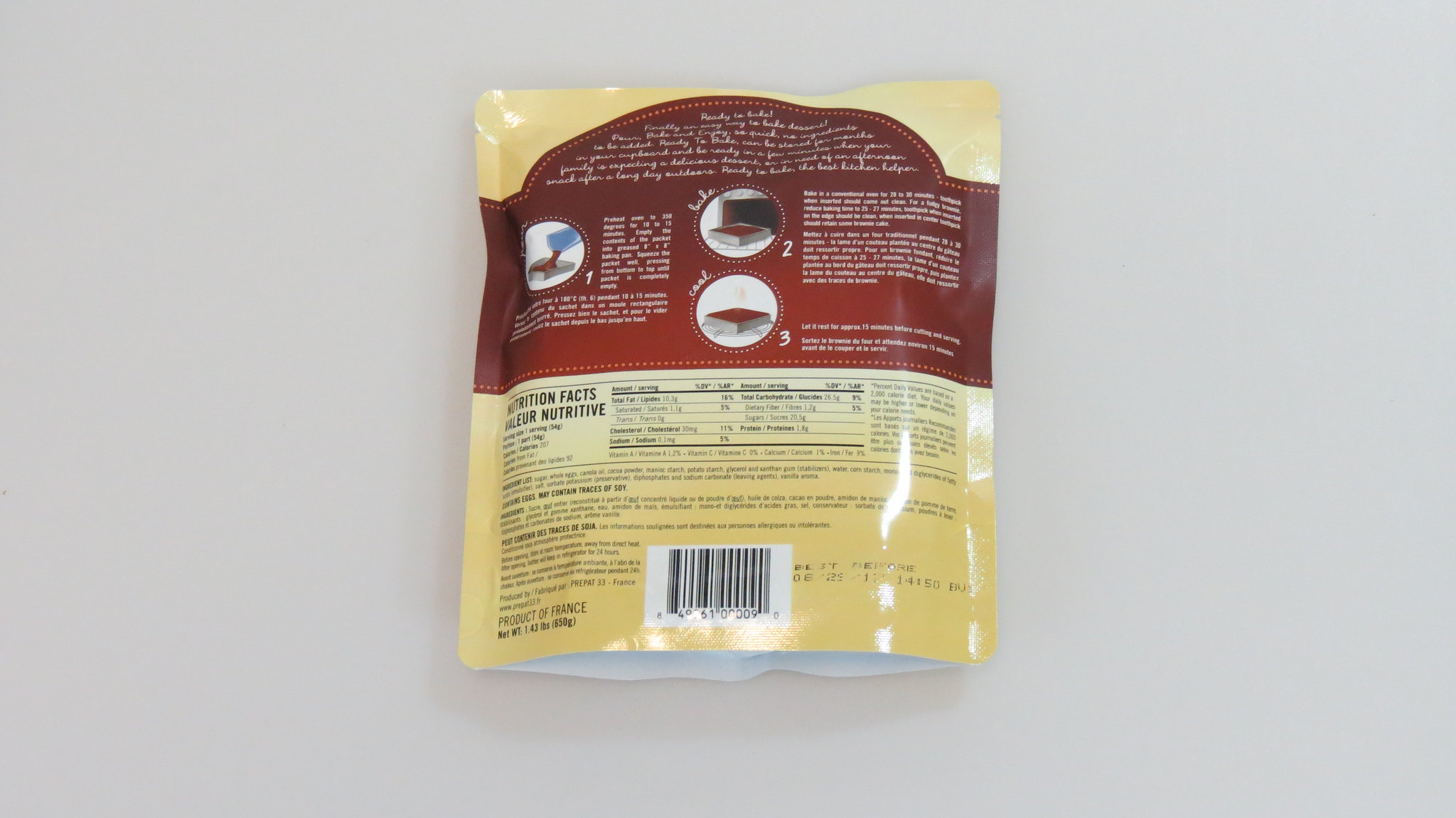The back of the package, most likely containing food, prominently displays nutrition facts, indicating its contents. The package is square-shaped and crafted from plastic, designed to stand upright with an opening at the bottom for stability. The main body of the package is tan, accented by a dark brown band at the top featuring unreadable cursive writing. 

Beneath this band, there are likely cooking instructions accompanied by three circular illustrations. The first circle shows a blue packet pouring what appears to be chocolate into a pan. The second circle depicts this chocolate mixture in a square pan with the word "Bake." The third circle is labeled "Cool" and suggests cooling the baked item.

While the package contains considerable text, it is small and difficult to read. It includes multilingual elements, particularly below the "Nutrition Facts" section where another language is present. At the bottom of the package is a black UPC symbol set against a white background.